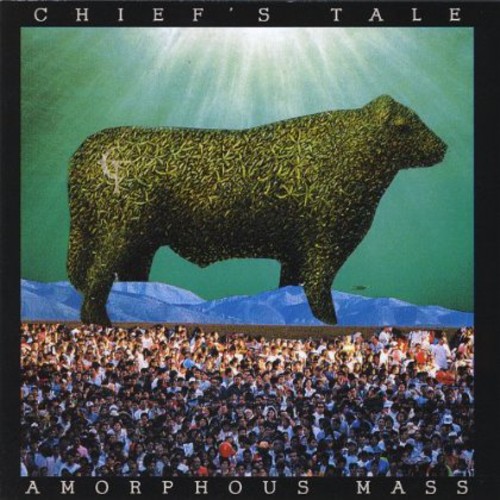This image features a surreal and abstract composition framed by a computerized black border. At the top, the words "Chief's Tail" are written in white capital letters on a black background, while the bottom displays the phrase "Amorphous Mass" in the same style. The central figure appears to be a large, fantastical creature that resembles a cow, though it might also be interpreted as a polar bear made of green plants, emphasizing its imaginative nature. This creature stands atop what seems to be blue-painted mountains. The sky behind it is unconventional, depicted in green with a shining sun highlighted in white. Below this strange creature, there's a striking contrast with a realistic photograph of a crowd of people, enhancing the overall sense of unusual and artistic interpretation that suggests it might be the cover of a book or a piece of conceptual art.